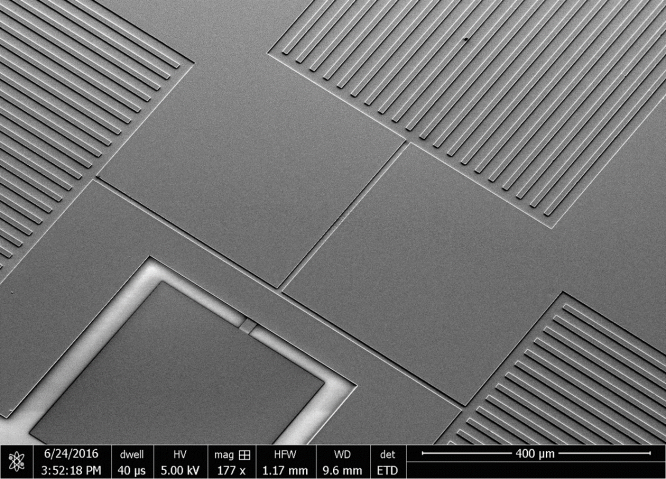The image is a horizontally oriented color photograph showcasing a fabricated grating and waveguide simulation for quantum force electronics. The primary focus is a textured gray board, divided into three main etched panels with vertical lines, positioned at the upper left, upper right, and lower right. These panels are interconnected by both vertical and horizontal etchings. The lower left of the board features an unconnected etched square with a central blank area, outlined in white. 

A segmented black bar stretches across the bottom edge of the image, marked by vertical white lines dividing the segments. The first segment on the left features a white atomic or nuclear logo, followed by the date "6-24-2016" and the timestamp "352.18 PM." Further segments display various scientific notations including "DWELL 40 ps," "HV 5.00 KV," and "mag," accompanied by a four-sectioned box and the annotation "177 X." Additional segments read "HPW 1.17 mm," "WD 9.6 mm," and "DET ETD." To the far right, there is a broken horizontal white line intersected by the number "400 um." The style of the image is representational realism with scientific notation and graphic design elements.